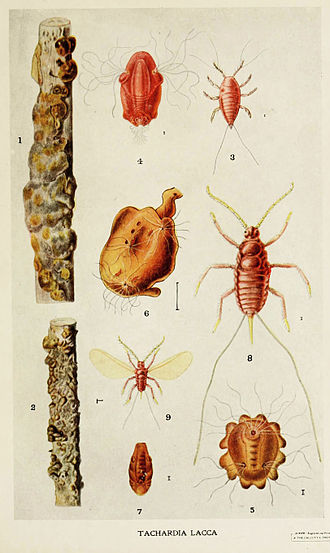This poster, set against a very light gray to white background, features a detailed diagram of various insects associated with two vertically positioned twigs on the left side. These twigs, appearing as light brown cylindrical branches, are covered with bumps and possibly show signs of insect activity. The insects are each numerically labeled from one to nine, accompanying the twigs along the right side.

At the top of the poster, the first insect is a red beetle, oval in shape, resembling a small spaceship, with no visible legs. Below it, a slimmer red beetle appears, featuring six legs and two antennae. The third insect is an undifferentiated blob-like shape, more orangish-brown in color. Following this is a larger dark red beetle, resembling the second but with a more pronounced body. The next figure is another dark red beetle, distinguished by two pale wings. Proceeding downward, two dark brown shapes appear—one oval and one with a curvy edge—perhaps hinting at different developmental stages or species variations. Concluding the sequence at the bottom, there is a shell-like structure followed by a crab-like beetle.

At the very bottom of the poster, the inscription "Tachardia lacca" is prominently printed in black uppercase letters, identifying the scientific context of the illustrated insects.